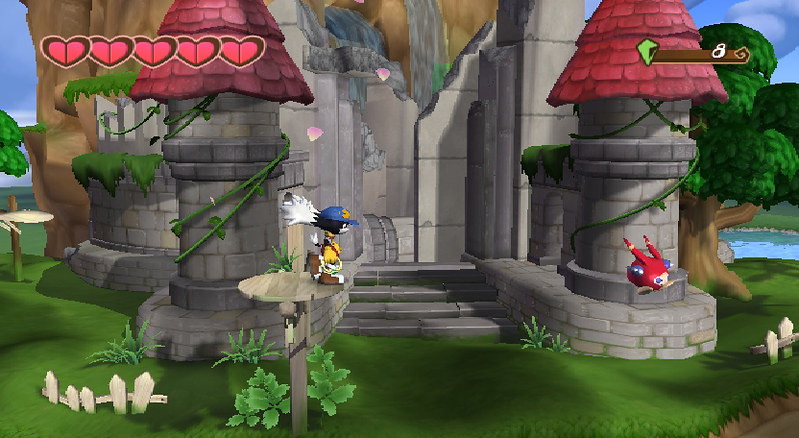The image features a close-up depiction of a video game scene centered around a majestic stone castle. The castle stands on a vividly green lawn, bordered by sections of a white picket fence flanking the entrance. Prominent stone turrets, adorned with lush green vines, frame the front entrance, adding to the castle's grand appearance. In the background, a serene body of water is visible, complemented by the rich greenery of numerous trees.

A red creature is seen gracefully flying in front of the castle. Observing this aerial display is another character, perched on a wooden platform beside the castle's front door. This character is distinguishable by his blue helmet and yellow shirt, attentively watching the red creature as it moves through the air.